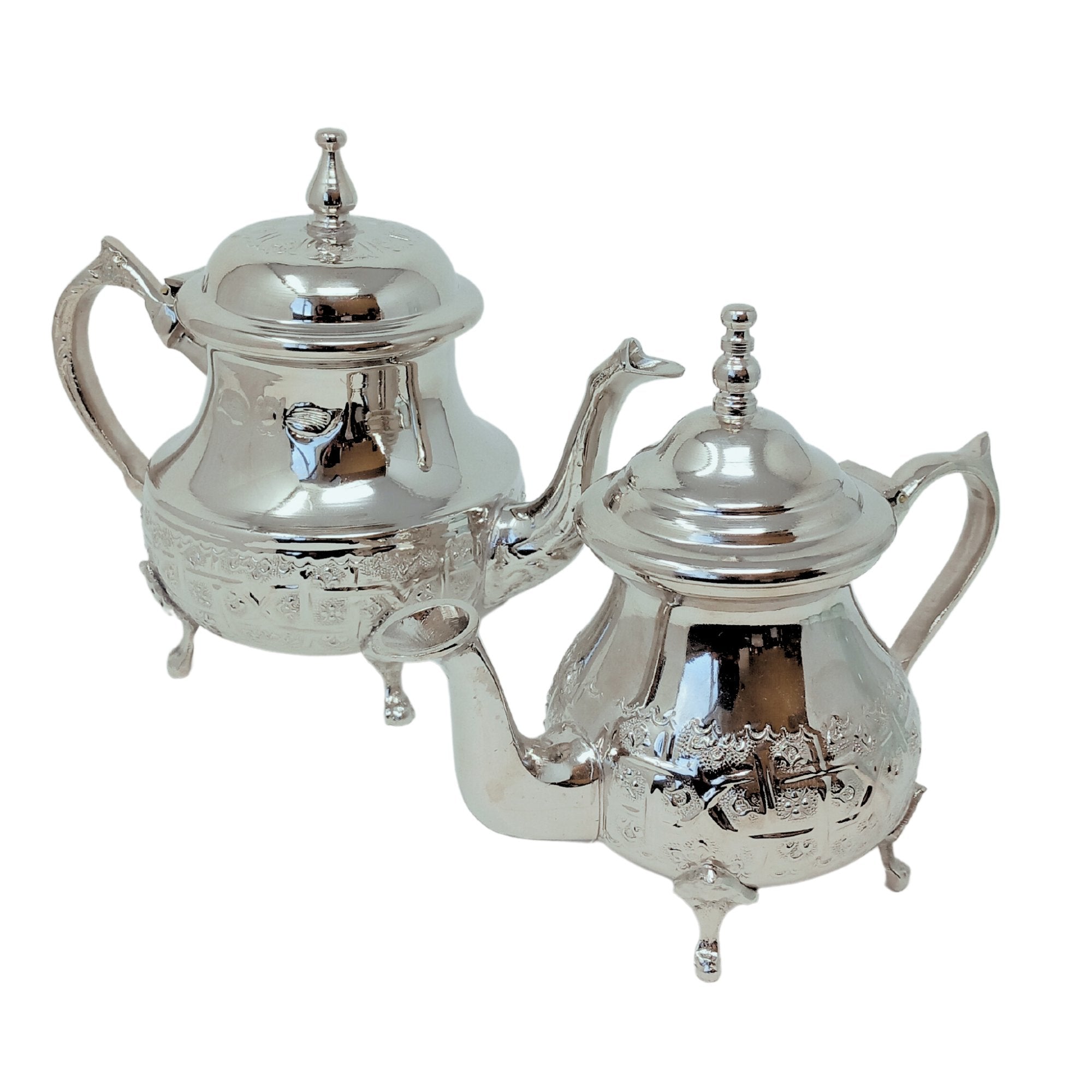This photograph showcases two sterling silver teapots, both exuding an elegant and classy appearance with their shiny, reflective surfaces. Positioned in the foreground, the teapot closer to the viewer features a slightly wider spout and a rounder shape compared to the teapot in the background, which boasts a larger, bell-shaped base. Each teapot sports its own unique lid design: the teapot in the foreground is adorned with a lid topped by four interlinked silver balls, while the background teapot has a one-piece gum or teardrop-shaped lid with a handle. Both teapots have intricately ornate patterning and differing engravings on their sides, adding to their sophisticated charm. The photograph suggests the presence of an unseen light source that enhances the reflectiveness and brilliance of these elegant silver pieces.